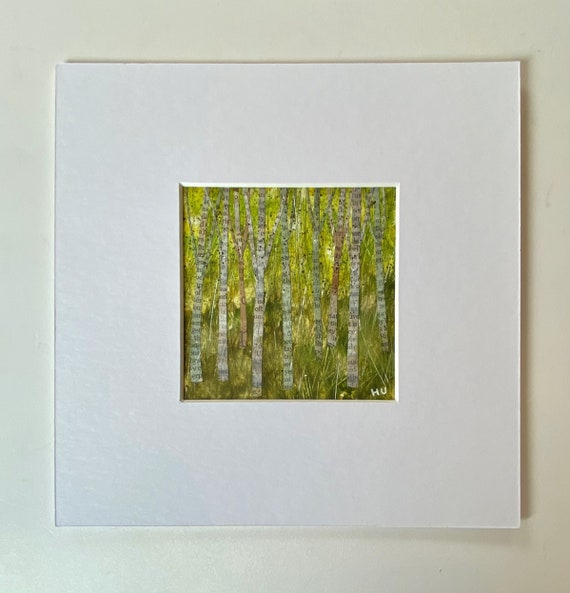The image is of a painting framed with a substantial white border, approximately six inches thick, and displayed against a cream or light gray wall. The painting within the frame depicts a dense forest featuring trunks of trees that resemble beech, birch, or aspen, characterized by their beige-brown or grayish bark with dark ring-like stripes ascending the trunks. The background of the artwork is filled with vibrant, lime-green foliage, indicating a rich, vegetative forest floor with bushes and branches. Light filters through the trees from the back, enhancing the lush greenery. Notably, no green foliage covers the trunks, and the top sections of the trees are not visible. The painting contains a small signature, "HU," in the bottom corner. The overall aesthetic of the artwork evokes a natural woodland scene, albeit with a somewhat generic feel.